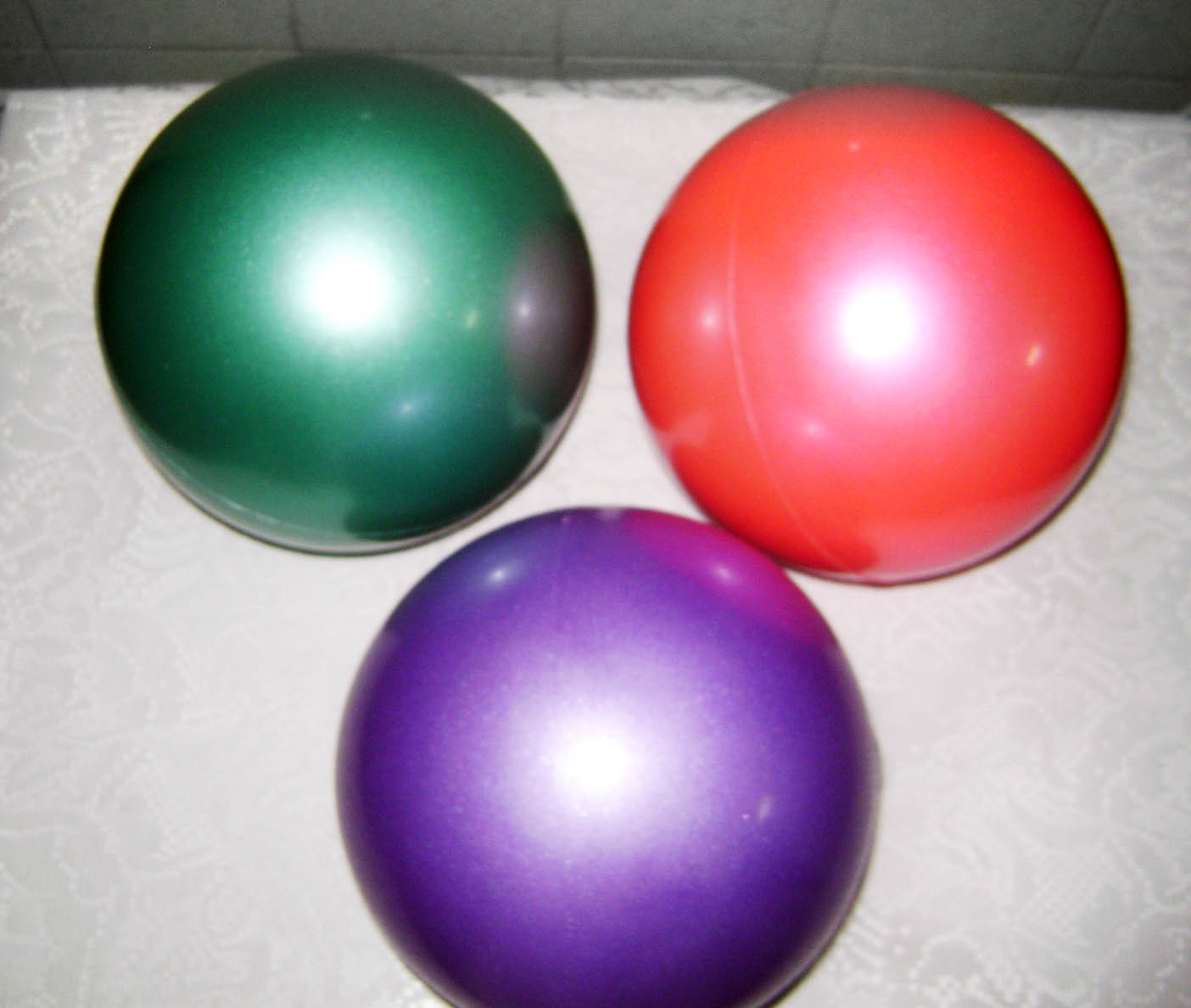This is an overhead color photograph showcasing three shiny, smooth rubber bouncy balls arranged in an upside down triangular formation on a light fabric background with a subtle, damask floral pattern. The balls, which occupy approximately 80% of the frame, are each equally sized and display prominent glare spots due to the lighting. The ball in the upper right corner is a blood orange-red with a large, bright glare spot in the middle. The ball on the upper left is a dark forest green, also featuring a nearly white glare spot at its center. Centered beneath these two is a purple ball with a more diffuse glare spot. The detailed fabric background transitions to a gray tiled wall near the top of the image, which appears to be in shadow. The lower part of the purple ball is slightly cut off at the edge of the frame.